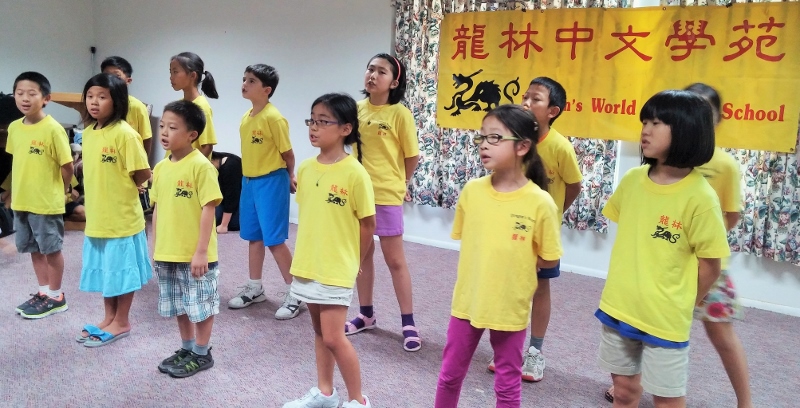The photograph depicts a group of twelve school-age children of Asian heritage, arranged in two rows of six. They are all wearing identical yellow shirts adorned with an Asian language script and a dragon logo on the chest. The children appear to be standing on a pink floor, possibly participating in a recital or singing, as suggested by their unified stance and expressions. They are dressed in various types of bottoms and shoes, and all have black hair. The background features a larger sign displaying the same Asian lettering and dragon logo, with the words "World School" partially visible in English beneath the Asian text. The setting appears to be indoors, characterized by white walls, and the entire scene is captured in a horizontal rectangular format. The colors present in the image include yellow, gold, red, black, gray, white, beige, pink, purple, blue, and aqua blue.